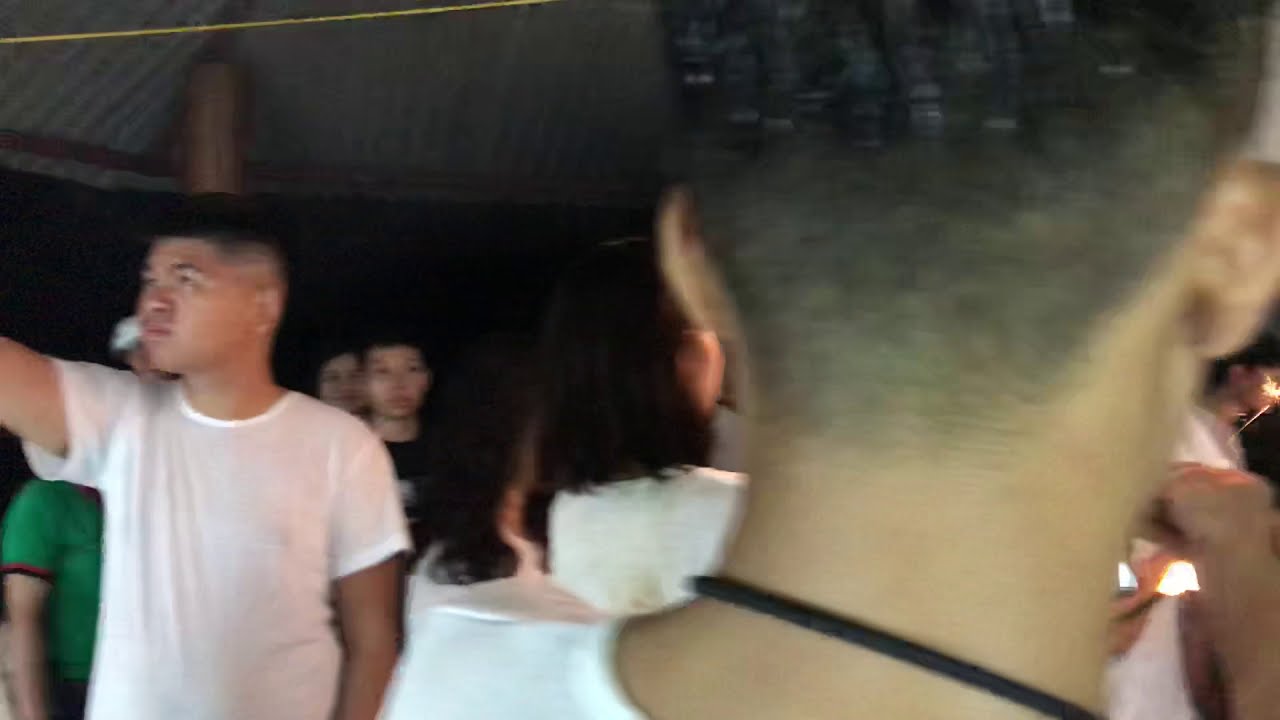The image captures a bustling scene of people standing inside a rustic building supported by log beams and topped with a corrugated metal roof. Dominating the right side of the frame is a man whose black hair is neatly trimmed. Only his neck and the back of his head are visible; he wears a white t-shirt and has a black strap around his neck, potentially for a camera or a necklace. To his left stands an Asian boy in a plain white t-shirt, with his right arm raised while he gazes outward. Partially obscured behind him is a person in a green t-shirt. Further in the background are glimpses of two individuals, likely a woman and a young boy, also wearing white. The gathering seems social, filled with conversation and interaction amongst the diverse group under the metal roof.